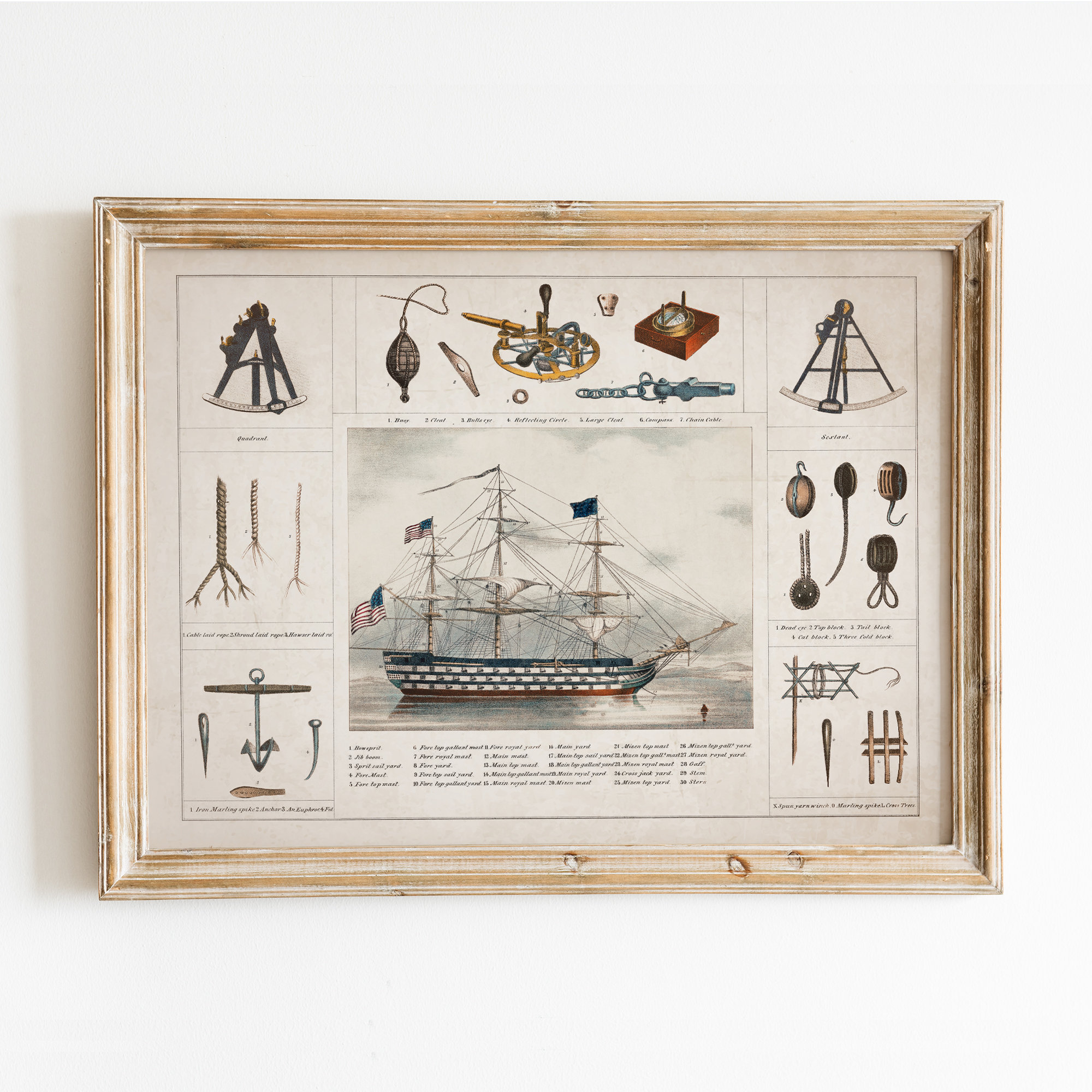The image depicts a close-up of a rectangular picture frame mounted on a light gray, off-white wall. The frame, made of a light brown wood, encloses a detailed illustration showcasing various components of a ship. At the center of the image is a ship adorned with several American flags and other nautical flags, with its sails pulled up and an intricate network of cables and ropes. Surrounding the central ship image are multiple smaller images: an anchor in the bottom left, various types of sextants, ropes, pulleys, and knots. These additional items are meticulously labeled, likely explaining their functions and placements on a ship. The photograph captures the scene in a well-lit indoor setting, emphasizing the clarity and detail of the intricate maritime illustration.